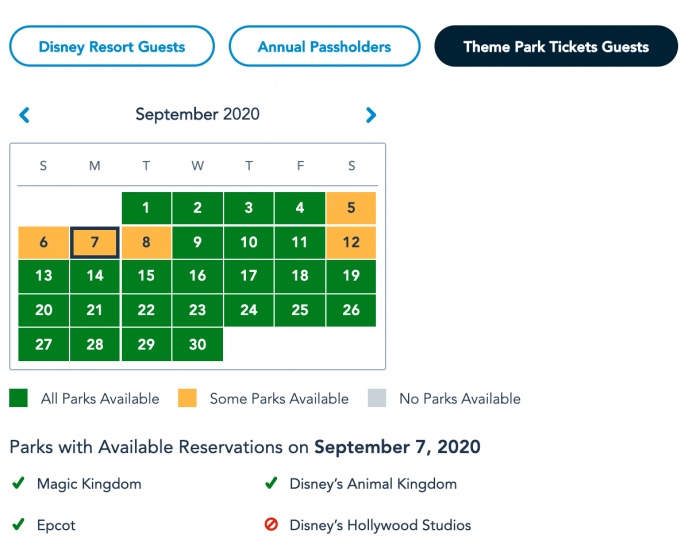This image captures a screenshot of a website, likely related to Disney park reservations. At the top of the page, there are three bubbles with text inside them. The bubble on the far left has a white background with blue text saying "Disney Resort Guests." The middle bubble has a similar design, stating "Annual Pass Holders." The bubble on the right is solid black with white text that reads "Theme Park Ticket Guests." Below these bubbles, a calendar for September 2020 is displayed, positioned towards the left side of the page. 

The calendar grid includes abbreviations for each day of the week: S, M, T, W, T, F, and S. Most of the dates on the calendar are shaded green. However, the 5th, 6th, 7th, 8th, and 12th are shaded yellow. A legend at the bottom explains the color coding: a green square indicates "all parks available," a yellow square signifies "some parks available," and a gray square would denote "no parks available."

Further down, there is a section titled "Parks with Available Reservations on September 7, 2020." It lists the availability of different Disney parks, highlighted with symbols and text. A green check mark is shown next to "Magic Kingdom," "Epcot," and "Disney's Animal Kingdom," indicating reservations are available for these parks. In contrast, a red cancel symbol is displayed next to "Disney's Hollywood Studios," signifying that reservations are not available for this park on the specified date.